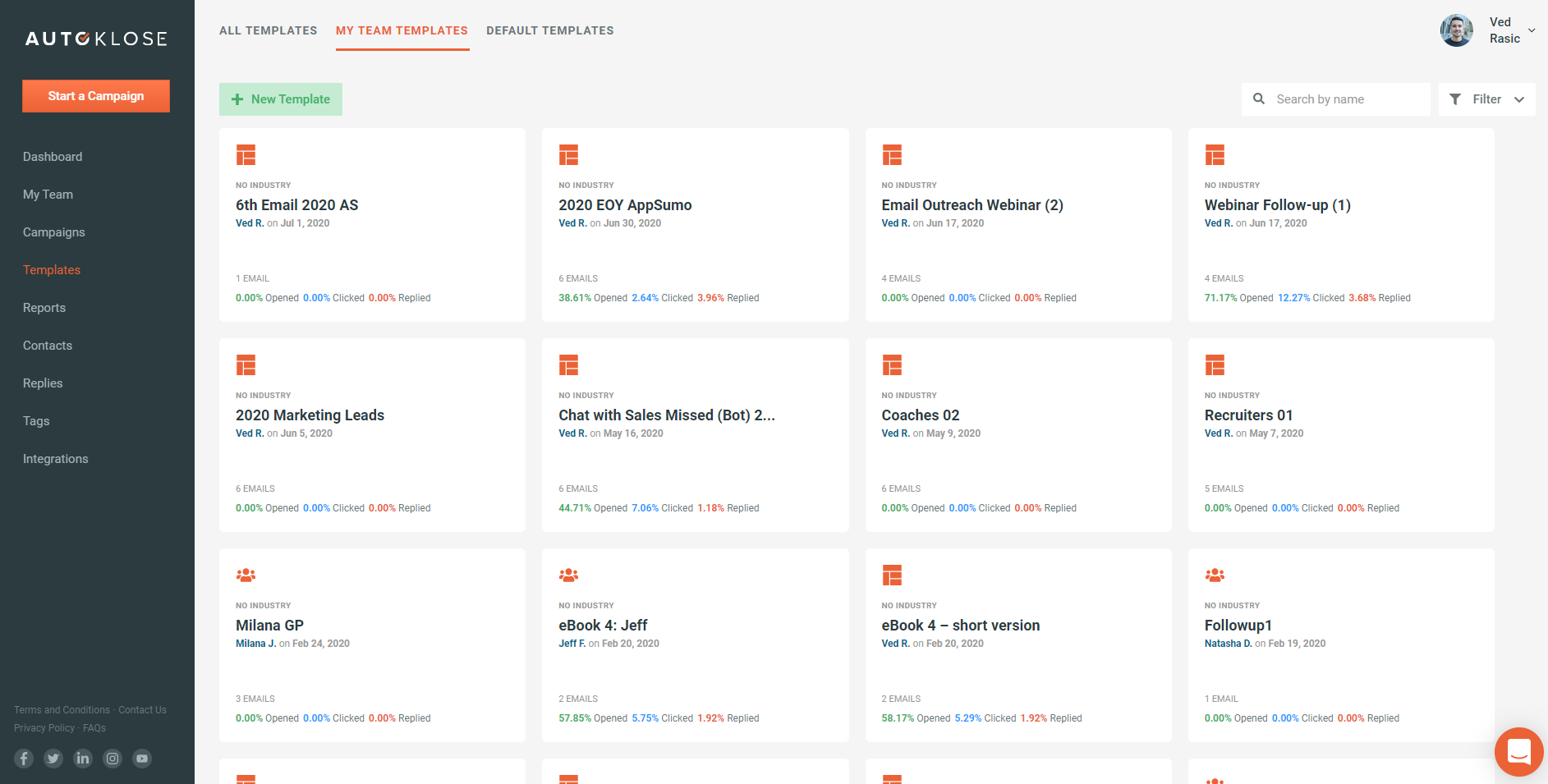The webpage features a user interface with a distinct layout. On the left, a vertical black sidebar extends from the top to the bottom. At the top of this sidebar, the text "Auto Klose" is prominently displayed, where "Klose" is uniquely spelled with a K. Just below this title, an orange button labeled "Start a Campaign" is situated. Further down the sidebar, there is a vertical menu with options stacked one below the other. The menu items are organized as follows: Dashboard, My Team, Campaigns, Templates, Reports, Contacts, Replies, Tags, and Integrations.

To the right of this sidebar, the main content area displays a white background. At the top of this section, there is a header with the text "All Templates," alongside two tabs: "My Team Templates," highlighted in red, and "Default Templates." Towards the far right corner of this header, a small circular profile picture of an individual appears, accompanied by an unreadable name.

The main white area of the screen is divided into a grid of templates, consisting of four columns across and three rows down, making a total of twelve blocks. Each block represents a different template, providing a neatly organized view of various template options.